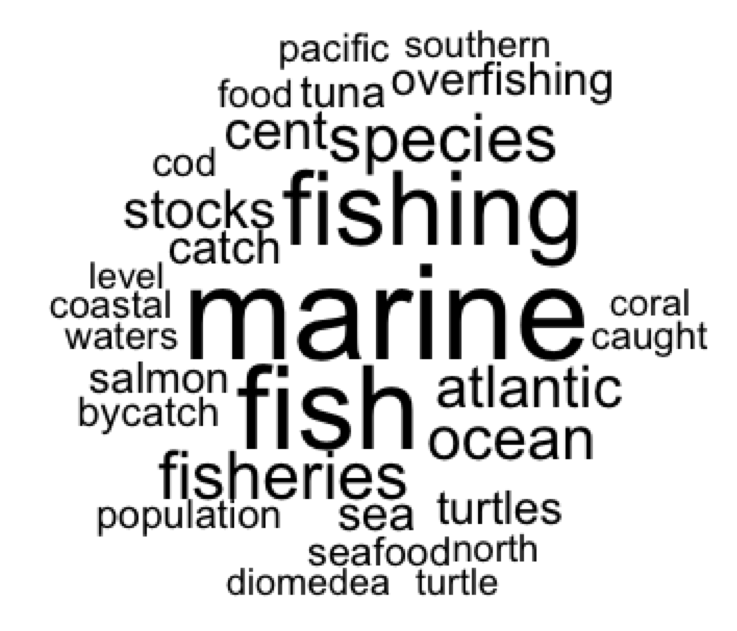The image is a detailed text cloud infographic, composed entirely of black lowercase words against a pure white background. The centerpiece features prominently large and bold words: "fishing," "marine," and "fish." Surrounding this central trio, the words gradually decrease in size, forming a kind of circular shape. Major terms related to the central theme of fishing and marine life are dispersed around the centerpiece, including "Pacific," "southern," "food," "tuna," "overfishing," "species," "cod," "stocks," "catch," "level," "coastal waters," "salmon," "bycatch," "fisheries," "population," "sea turtles," "seafood," "north," "diomedia," "turtle," "Atlantic Ocean," "coral," and "caught." The larger words in the center emphasize the primary focus of the infographic, while the surrounding smaller words provide a detailed context related to fishing and marine ecosystems.